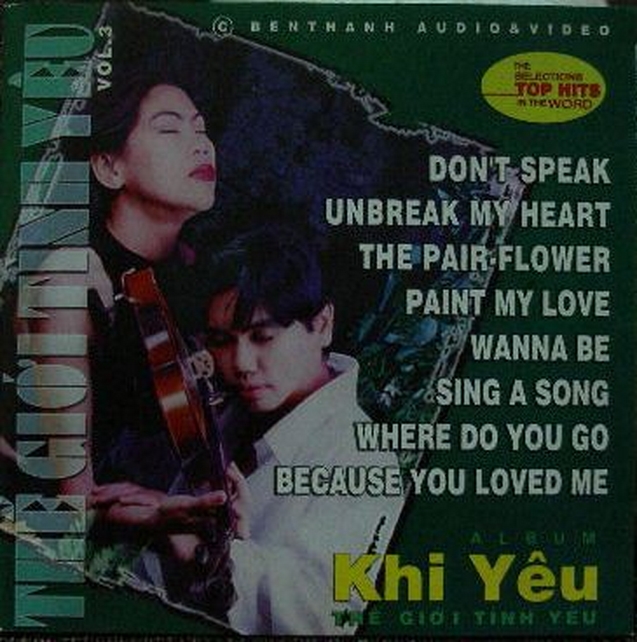This image is a highly detailed record cover. At the top of the cover, the text reads "Copyright, Menthon Audio and Video." Just below, there is a prominent yellow oval shape with the title "Selections: Top Hits in the World." On the right side of the cover, we see a list of songs: "Don't Speak," "Unbreak My Heart," "The Pear Flower," "Paint My Love," "Wannabe," "Sing a Song," "Where Do You Go," and "Because You Love Me." Additionally, the album is noted to be by "Kai Yu" and "The Goi Tin Yu," volume three. 

The central image features a woman with closed eyes, red lipstick, and an upward gaze, tenderly holding a violin. Next to her is a young boy in a white shirt, who is touching the wrist of her hand that is holding the violin. His head is resting on her shoulder, and his eyes are also closed, which suggests a serene or intimate moment between them. On the left side, vertically and sideways, the text reads "The Goi Tin Yu, Volume Three."